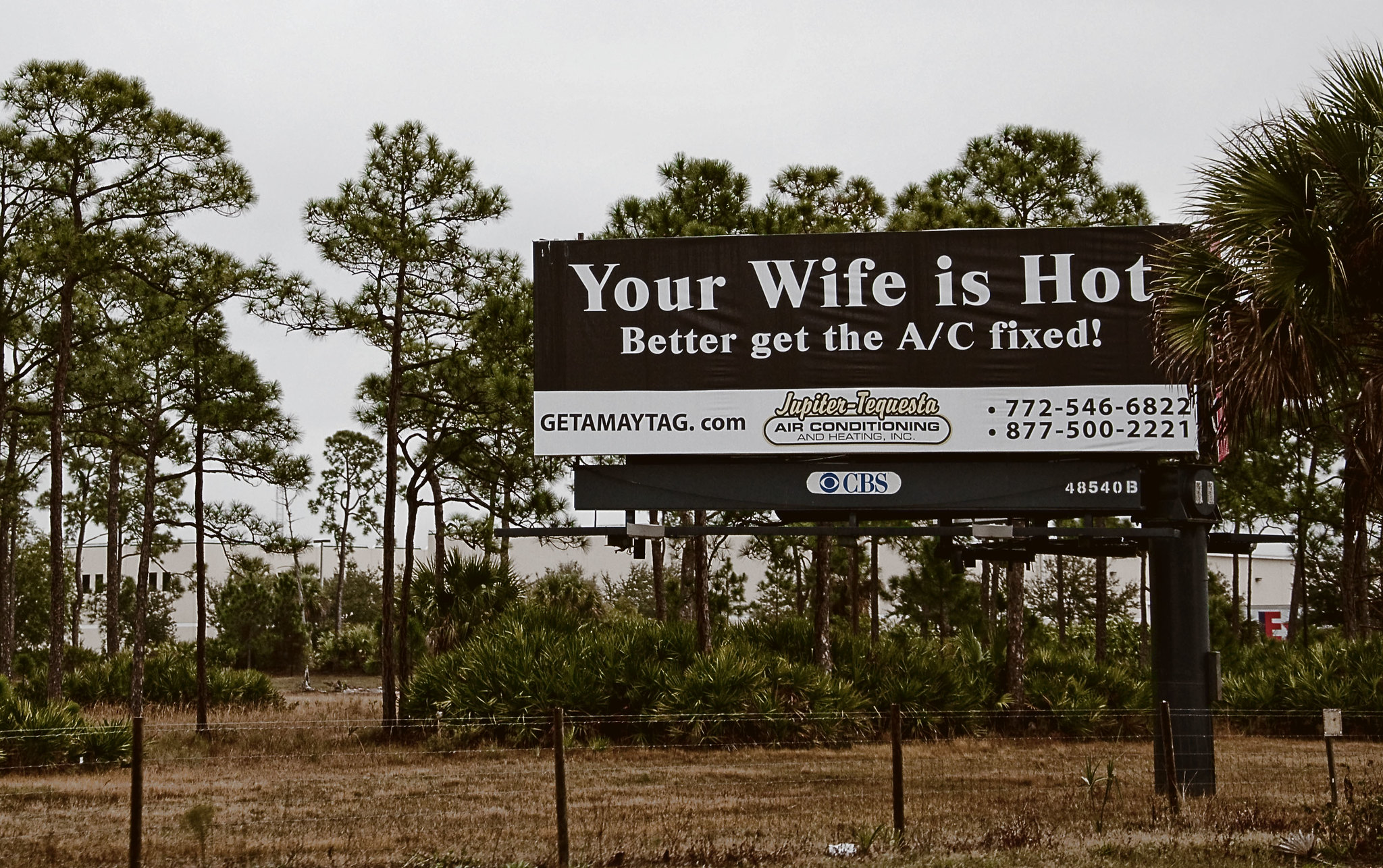The photograph captures a somewhat humorous billboard set against a gray, overcast sky. The background features a mix of sparse pine trees and palm-like bushes, suggesting a subtropical or warmer climate. To the right of this foliage, a singular palm tree stands prominently. A white building is visible through the trees, and a wire fence runs along the foreground, adding a touch of structure to the scene.

The billboard itself has a compelling design. The upper portion features a black background with bold white text that reads, "Your wife is hot. Better get the AC fixed!" Below this eye-catching message, another section with a white background provides more information. It advertises a website, "getamaytag.com," and promotes the business, "Jupiter-Tequesta Air Conditioning and Heating, Inc." Two phone numbers are listed for contact: 772-546-6822 and 877-500-2221. Additionally, the sign includes the text "CBS" and the code "4854-0B" on the lower right-hand side, likely indicating some form of identification or attribution. 

The overall scene is a juxtaposition of natural and man-made elements, and the billboard's humorous message adds a lighthearted twist to the otherwise gloomy backdrop.